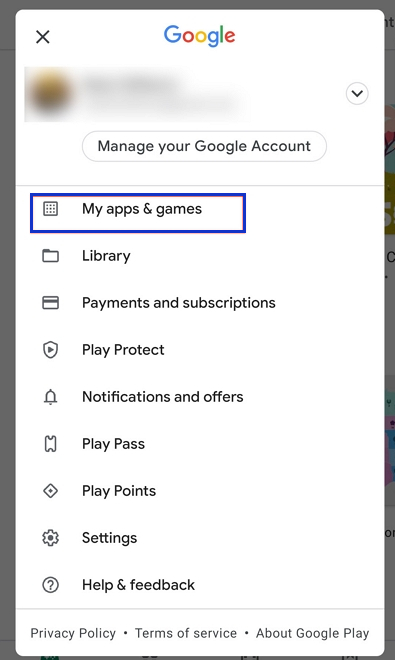This is a screenshot of the pop-up menu on the Google Play Store. The background is dimmed and partially obscured by a prominent white overlay box. At the very top of the box is the title "Google," presented in Google's signature colors. To the left of the title is a black X icon, presumably for closing the menu. Below the title, there is some blurred-out information for privacy reasons, with a drop-down arrow to its right for expanding additional options.

Further down, there is a button labeled "Manage your Google Account," written in black. The text on the page features a mix of black and grayish fonts. Various categories are listed, each with corresponding icons. The first visible category, "My apps & games," is highlighted with a blue outline.

At the bottom of the menu, there are three additional options for navigation: "Privacy Policy," "Terms of Service," and "About Google Play."